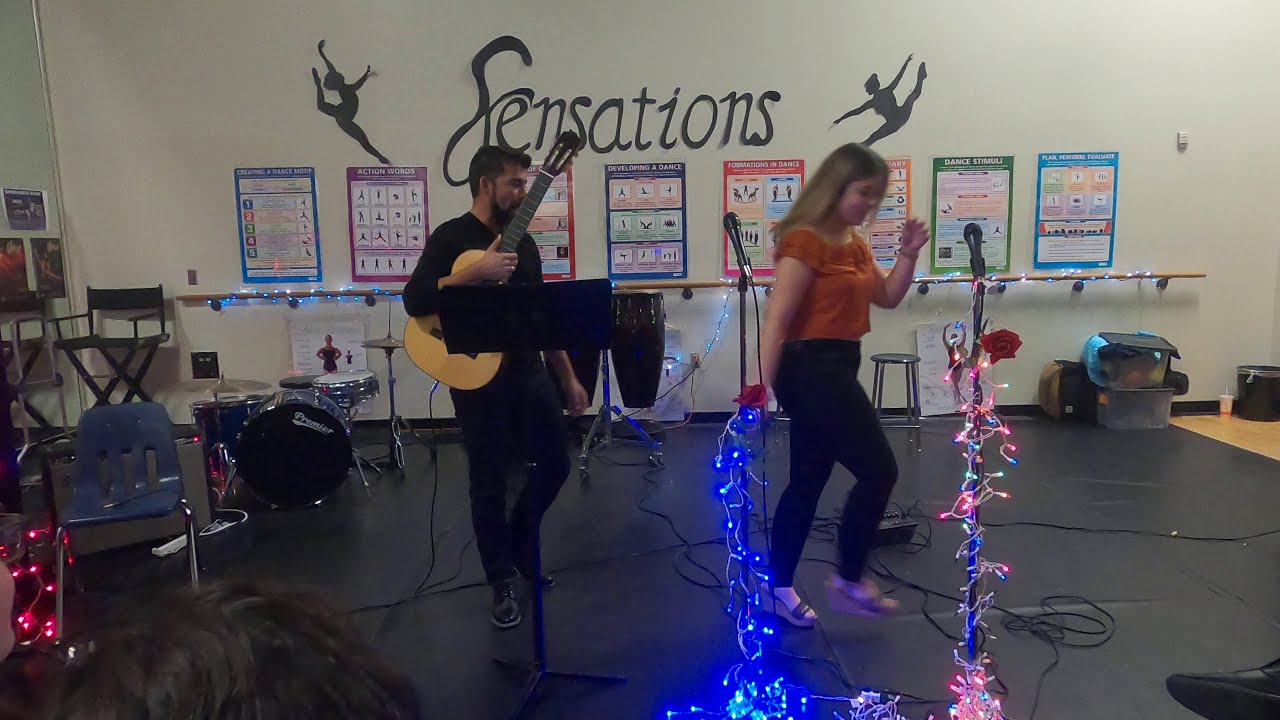This horizontally aligned rectangular image, taken indoors, showcases a performance-like setting with two people positioned in the foreground on a dark gray tile floor, resembling a stage. Dominating the white background wall is the word "Sensations" in black letters, flanked by silhouettes of dancers or gymnasts. Below this, approximately seven or eight posters display various dance information and positions. 

To the left, a light brown-skinned man, dressed entirely in black, holds a tan guitar in his right hand, his short dark hair and facial hair clearly visible. To his right, a woman in an orange short-sleeved top and black pants is mid-dance, her right foot elevated and her left foot grounded, demonstrating a graceful pose with her elbow bent. She sports long brown hair and sandals. 

In front of both performers, several microphones on stands are adorned with colorful lights: one with blue lights, another with multicolored ones. A blue plastic chair and a drum set are visible to the left, while a railing against the wall, wrapped in additional lights, amplifies the festive atmosphere. At the bottom left corner of the image, the top of someone’s brown hair, presumably an audience member, is just visible, capturing their attention on the performing duo. The room is well-lit, adding vivid clarity to the scene.